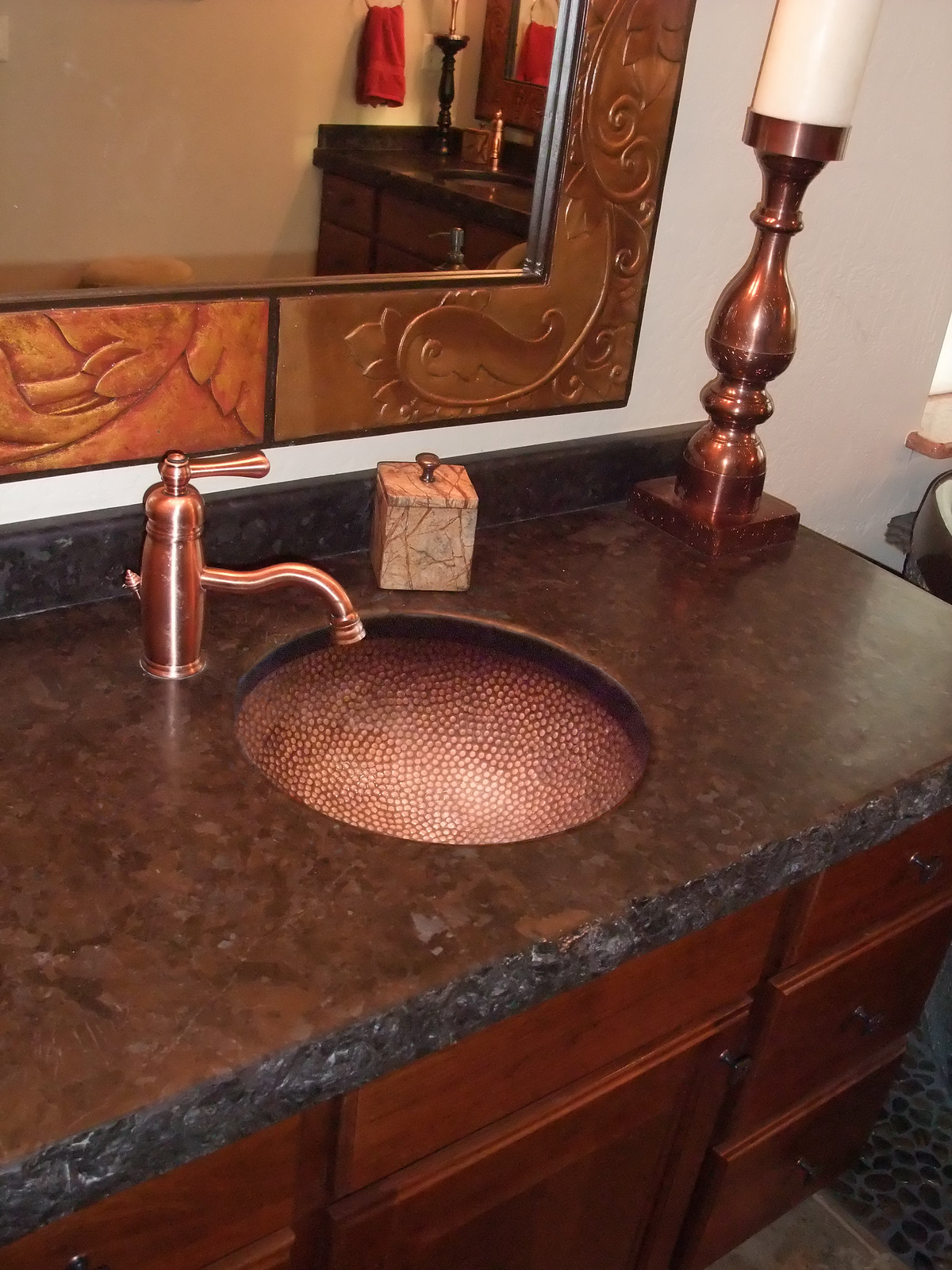This photograph showcases an opulent bathroom setting, featuring a striking centerpiece—a luxurious, bowl-shaped sink with a gold finish. It rests on an elaborate marble or granite countertop that exhibits a rich, brown hue on the surface and appears to transition into black along the sides, possibly due to a reflective property. This intricate countertop is complemented by an elegant brass faucet, extending from a cylindrical base and topped with a rounded knob.

Adjacent to the sink, on the right corner of the countertop, stands a distinctive lamp, adding to the room's sophisticated ambiance. Below, a series of drawers and cabinets offer functional storage solutions, seamlessly blending with the lavish decor.

A grand mirror, encased in a golden frame adorned with intricate etchings of marine life such as whales, dominates the background. This heavy and ornate mirror reflects another part of the bathroom, revealing a second sink. A red hand towel, hanging in the reflection, adds a pop of color and further enriches the scene.

The flooring beneath features a dual design: a sleek, blackish-gray tile alongside a strikingly patterned surface with sporadic black and white circular motifs, enhancing the room's overall elegance. This attention to detail and the opulent fixtures suggest that the room is indeed a very fancy bathroom.